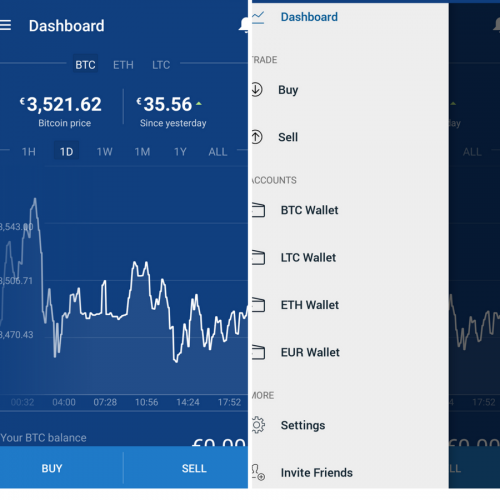A detailed caption for the image:

The image showcases a smartphone screen displaying a cryptocurrency management dashboard. On the left, there is a blue panel labeled "Dashboard." At the top of the screen, the cryptocurrencies BTC (Bitcoin), ETH (Ethereum), and LTC (Litecoin) are listed. BTC is currently selected, showing its price as €3,521.62, with an increase of €35.56 since the previous day. Below, there are options to view the price fluctuations over different time periods (one hour, day, week, month, year, and all time), with the day chart currently selected. A graph illustrating the price changes throughout the day is also visible. At the bottom, there are light blue buttons for buying and selling Bitcoin.

To the right, partially visible, seems to be a second screenshot, possibly stitched together with the first. This side also shows the dashboard but includes additional options like Trade, Buy & Sell, and Accounts, which are partially cut off. Visible components include BTC Wallet, LTC Wallet, ETH Wallet, and EUR Wallet. Further down, there are options for Settings and Invite Friends. Another graph appears to be truncated at the far right, suggesting it is part of the overlay panel from the left screenshot, offering more navigational and functional options for users.